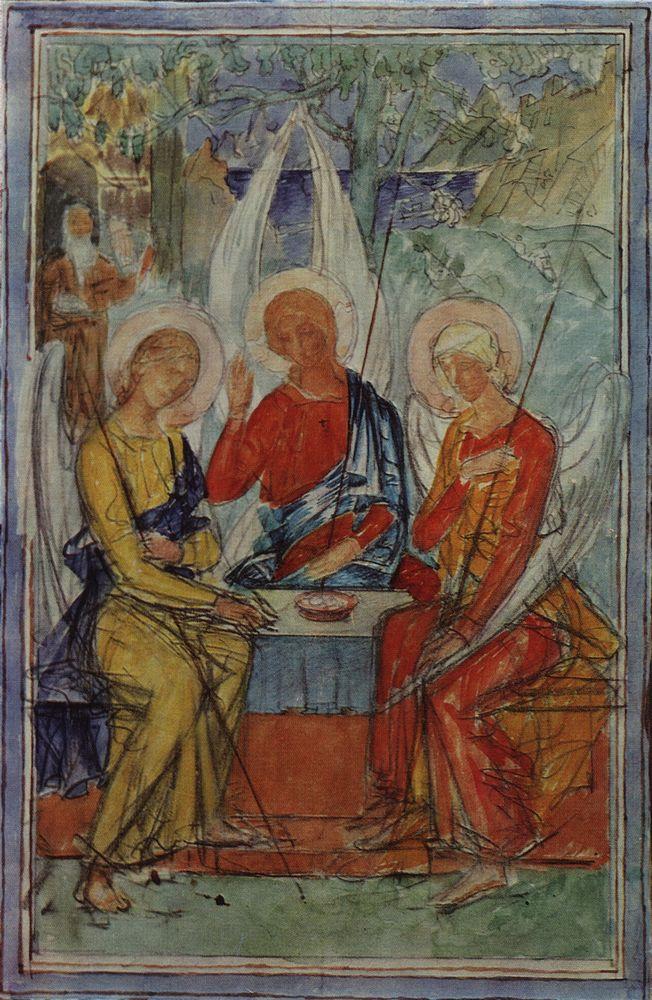The image portrays a detailed and vividly colored artwork featuring three angelic figures, seated around a table with a central red bowl, creating an atmosphere reminiscent of a sacred gathering. Each angel has distinct attire and wings: the angel on the left wears a yellow outfit complemented by a blue sash and a halo, her wings arched downward. The central angel, in red with a blue sash, stands out by having upward-pointing wings, indicating a unique status among the trio. The rightmost angel also wears red, paired with an orange sash and a halo, her wings similar to the left angel's, arcing downward.

In the background, against a natural landscape of green trees, mountains, and a serene lake, stands an elderly man with a white beard, dressed in a brown robe. His presence adds a profound, almost biblical layer to the scene, suggesting figures like Moses or Noah. Surrounding details, though sketchy, include cliffs, rocks, and a castle-like structure, heightening the sense of a fantastical, yet religious tableau. Despite its sketchy art style, the vivid colors and implicit spiritual symbolism render a complex and compelling visual narrative.